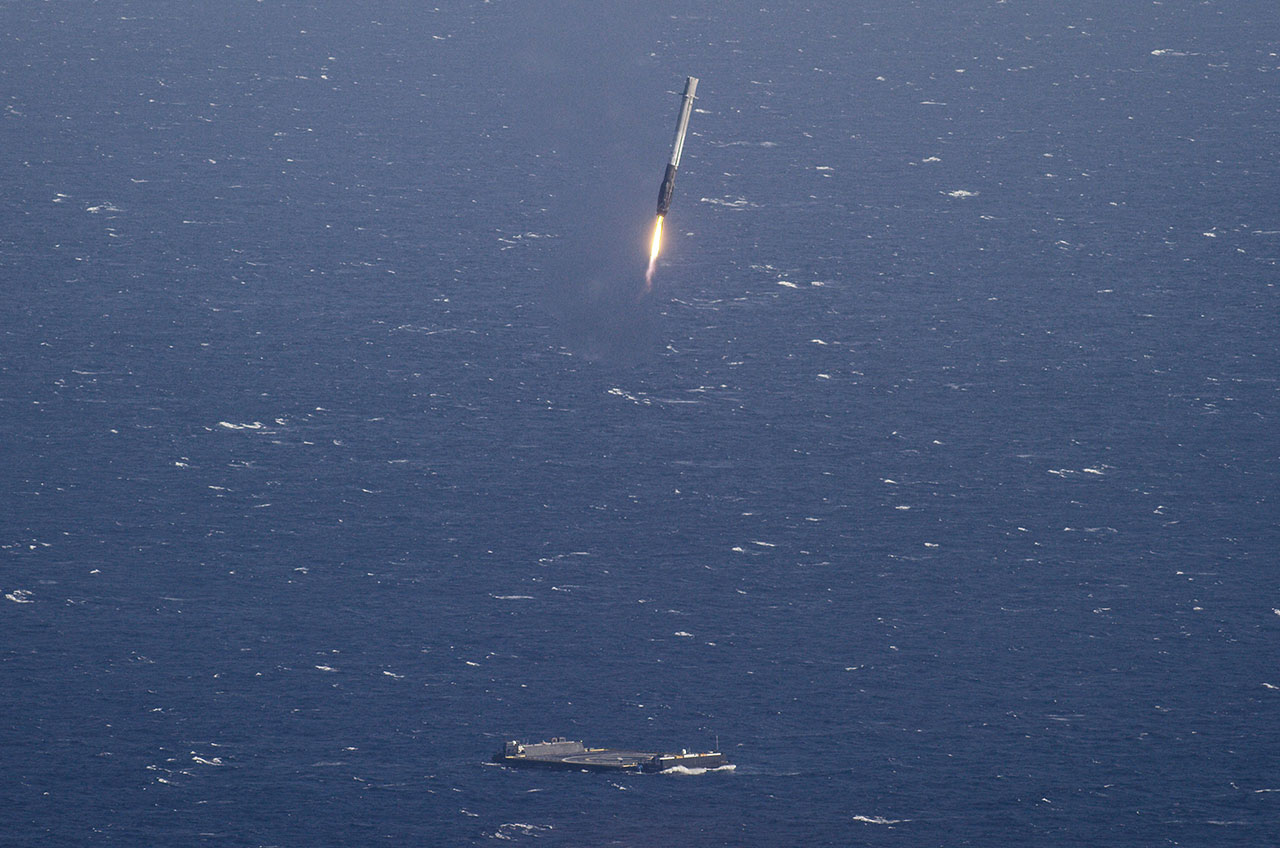The photograph captures a dramatic scene in a vast, dark blue ocean with a hazy gradient, transitioning to a grayish hue near the top of the image. The ocean appears mostly calm with subtle wave breakers distributed throughout. At the bottom center of the image lies a small, black platform, indicating a launch platform, which looks tiny in comparison to the expansive body of water. Emerging from the platform is a light gray rocket with fire spewing from its base, distorting the air around it with heat blur. The rocket, slightly angled to the right of the vertical axis, appears to be taking off, enveloped by the open sea.